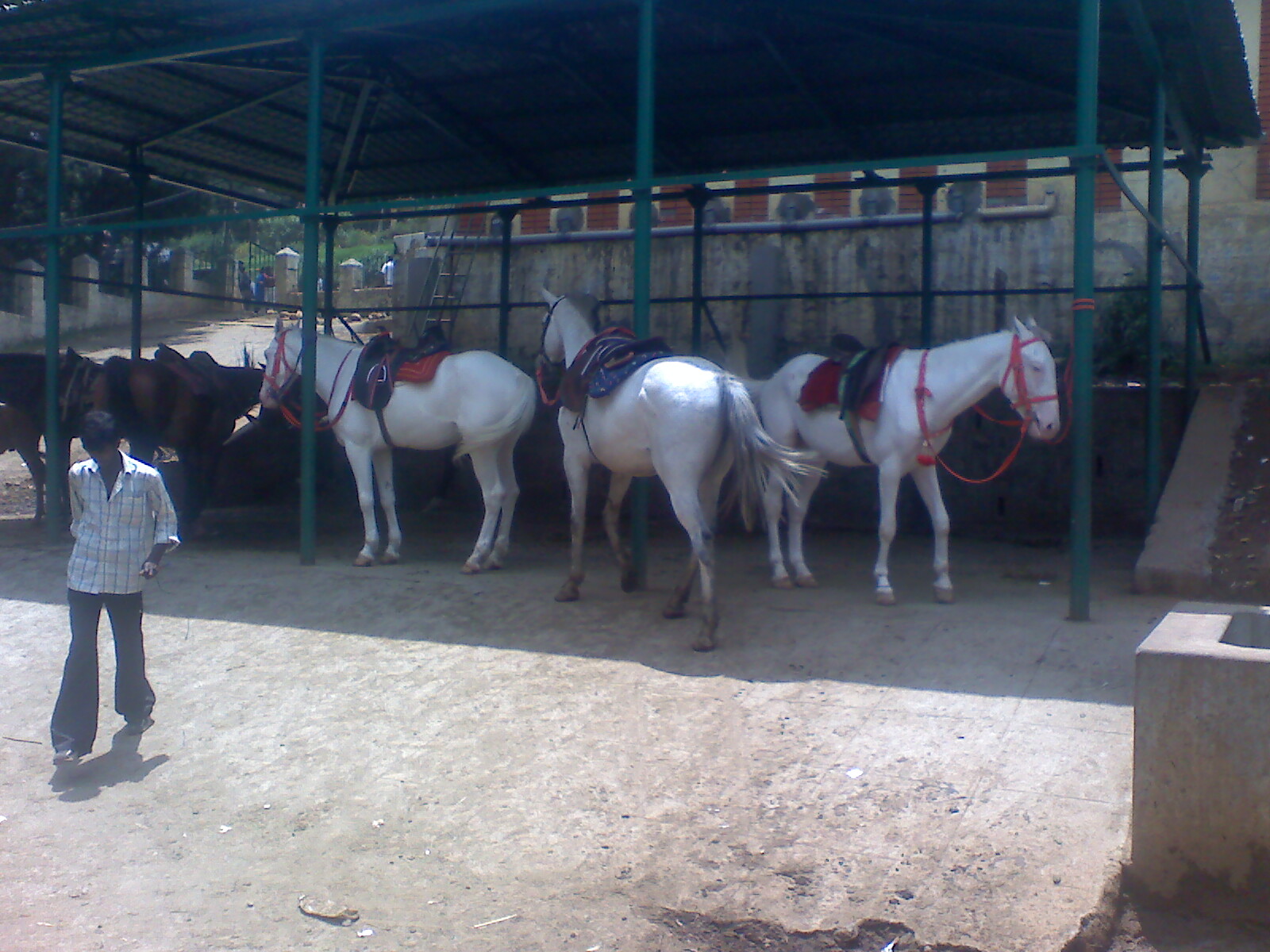This photograph features a rural fair setting with an open-air stable identifiable by its structure of green metal poles supporting a raised roof, possibly thatched or corrugated metal, that arches slightly in the center. The sides of the stable are constructed from the same green material, offering a clear view through to the other side, which showcases a yellow, blue, and red banner running along the top, enhancing the festive atmosphere.

In the forefront, three white horses stand prominently, each adorned with bright, colorful saddles—a red one on the left and right horses, and a blue on the middle one—flanked by matching red bridles and harnesses. The horse on the right faces towards the camera, while the other two face away.

To the left side of the image, a man with short black hair, possibly of East Indian descent, dressed in a white shirt with blue cross-striped patterns, bell-bottom jeans, and a bow cap—depicted walking towards the camera. Behind him are more horses, predominantly brown, scattered towards the back of the stable.

The ground beneath the stable is concrete, transitioning to a dirt path where the man walks. In the background to the right, there are cement structures that appear to be part of the fairground's layout, adding depth and context to the bustling setting.